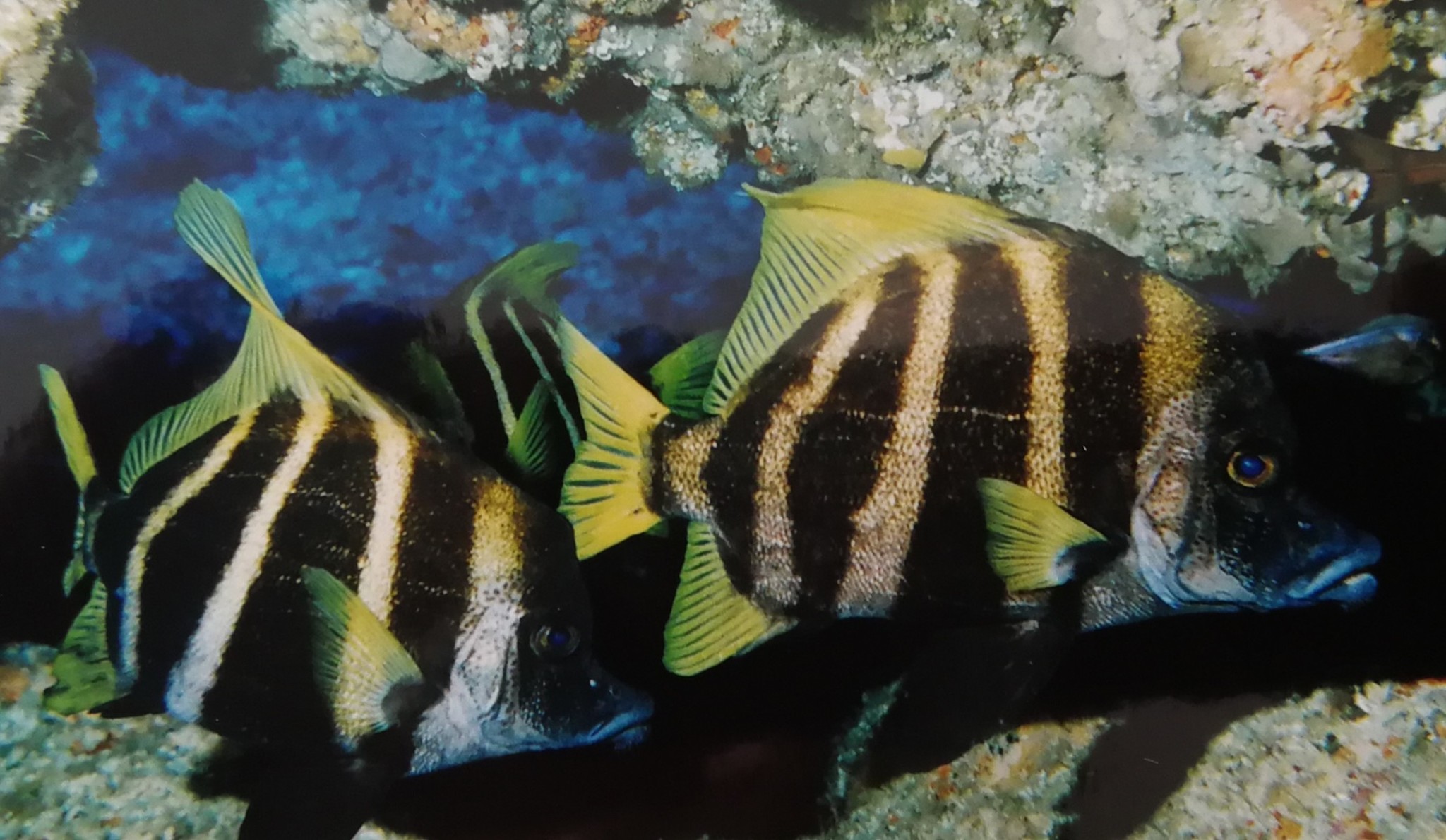In this zoomed-in underwater image, we see three striped fish, prominently featuring black and white stripes with the black stripes being more pronounced and wider. The fish possess striking yellow and green fins; the color gradation transitions from yellow near their bodies to green towards the edges of their fins and tails. The fish also exhibit large gold eyes and a distinct face, with a protruding nose reminiscent of a duck bill, and a mouth at the tip. They are seen moving towards the right.

Surrounding the fish is a colorful reef composed of rough, conglomerated rocks. The rocks are predominantly gray with specks of orange, red, and even some green. In the background, there are patches of dark blue, likely representing either more underwater rocks or the water itself, adding depth and contrast to the scene. The overall setting suggests a vibrant and dynamic underwater environment, teeming with life and geological variety.